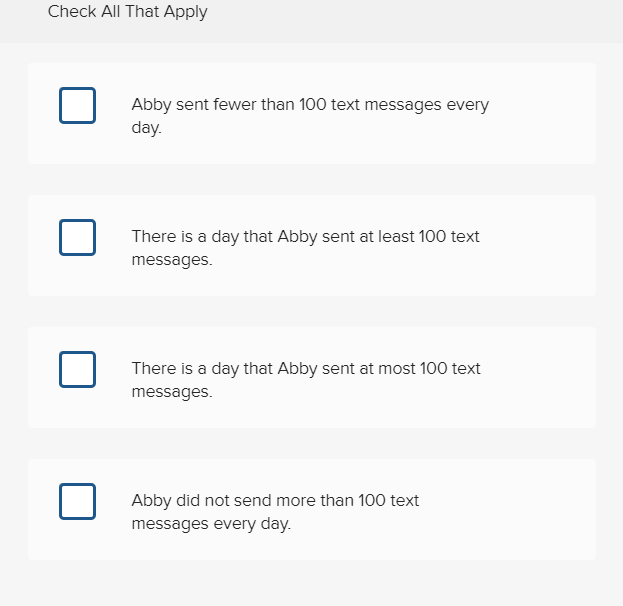The image is a rectangular interface with a light gray background. It features a header section at the top, which is a medium gray and contains black text in a basic sans-serif font. The header text, "Check All That Apply," is not bolded and follows title case formatting.

Beneath the header, the light gray background continues, hosting four distinct rectangular sections. Each section has a very light gray background, further separated by tick boxes located to their left. These tick boxes are outlined in navy blue, with slightly rounded but predominantly square corners. The interiors of the tick boxes are white and currently none of them are checked.

The tick boxes are accompanied by text descriptions in gray font:
1. "Abby sent fewer than 100 text messages every day."
2. "There is a day that Abby sent at least 100 text messages."
3. "There is a day that Abby sent at most 100 text messages."
4. "Abby did not send more than 100 text messages a day."

The text inside the tick boxes sections is smaller in size compared to the header, approximately 80% of its size, and these sections are centered within the image.

Additionally, the header text begins with a small indentation akin to a tab space. The interface has a significant light gray margin at the bottom, about double the size of the margin at the top, providing a balanced design.